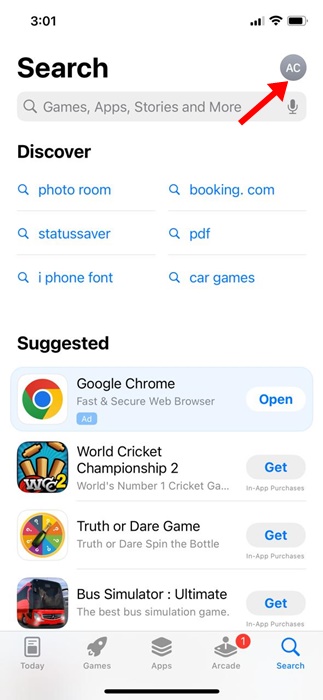Screenshot of a Mobile Device Search Results Page at 3:01 PM

The image is a screenshot taken from a mobile device displaying the results of a search. At the upper-left corner, the time is shown as 3:01 PM. Directly beneath the time, the word "Search" is written in black text. Below this, there is a search bar with a search icon, featuring the placeholder text "Games, apps, stories, and more" on a light gray background.

Beneath the search bar, the word "Discover" appears in black text, followed by six search suggestions written in blue text. Further down, "Suggested" is displayed in black, leading into a section of suggested applications. This section is organized into four rows, each displaying a different application icon on the left.

The first row features the Google Chrome application, followed by "World Cricket Champion 2," the "Truth or Dare" game, and lastly, "Boss Simulator Ultimate." Each application entry includes its respective icon and name, providing a clear and organized view of suggested apps based on the search query.